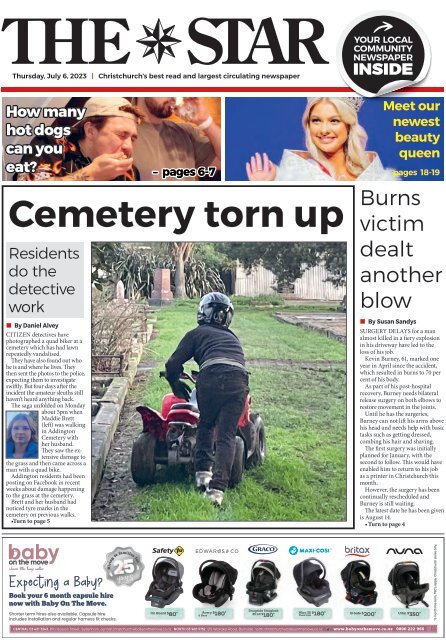Front Page of The Star - July 6, 2023 Edition:

- **Masthead**: "The Star" with a 3D star graphic placed between 'The' and 'Star.' Below, in a circular icon, the phrase "Your Local Community Newspaper" is prominently displayed.
- **Publication Date**: Thursday, July 6, 2023.
- **Tagline**: "Christ Church's Best Read and Largest Circulating Newspaper."

### Main Headlines:

1. **How Many Dogs Can You Eat?** 
   - **Images**: Features a photograph of two men eating.
   - **Article**: Details and continuation found on pages 6 and 7.
   
2. **Meet Our Newest Beauty Queen**
   - **Images**: Showcases an individual crowned as a beauty queen.
   - **Article**: Further details available on pages 18 through 19.
   
3. **Cemetery Torn Up**
   - **Images**: Depicts a child riding a four-wheeler, implying the activity takes place in a cemetery.
   - **Headline**: "Residents Do the Detective Work" by Daniel Avey.
   - **Article**: Consists of approximately three paragraphs on the front page, continuing onto page 5.

4. **Burn Victims Dealt Another Blow**
   - **Images**: None specified.
   - **Headline**: By Susan Sandus.
   - **Article**: Features around four to five paragraphs on the front page, with further details continuing on page 4.

### Advertisement:

- **Bottom of the Page**: An advertisement for "Baby on the Move," showcasing various baby carriers.